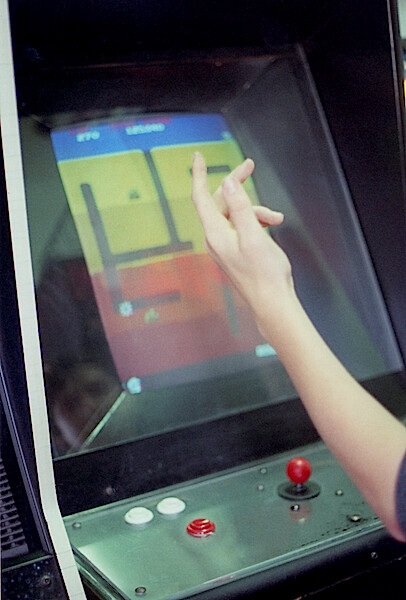This image features a close-up of a vintage arcade game cabinet, angled diagonally to reveal a sliver of another cabinet on the left. The arcade machine itself has a green and black exterior. The screen displays a classic game with a layout reminiscent of pong or a tunnel-digging game like Dig Dug. The screen is divided into five horizontal color bands: blue at the top, transitioning through two shades of yellow, then orange, and finally red at the bottom, with black lines creating a grid or tunnels.

In front of the screen, a fully extended left forearm is visible, likely belonging to a young male wearing a brown or gray short-sleeved shirt. His shirt is partially obscured by the angle, but the gesture of his hand—three fingers extended, suggesting frustration or exclamation—is clear. The control panel near his elbow features a red ball joystick centrally positioned, flanked by two white buttons to the left and a red button below the rightmost white button.

Reflected on the screen is the faint image of the person playing, adding a layer of interaction to the image. The overall scene captures the intense, nostalgic engagement typical of classic arcade gaming.